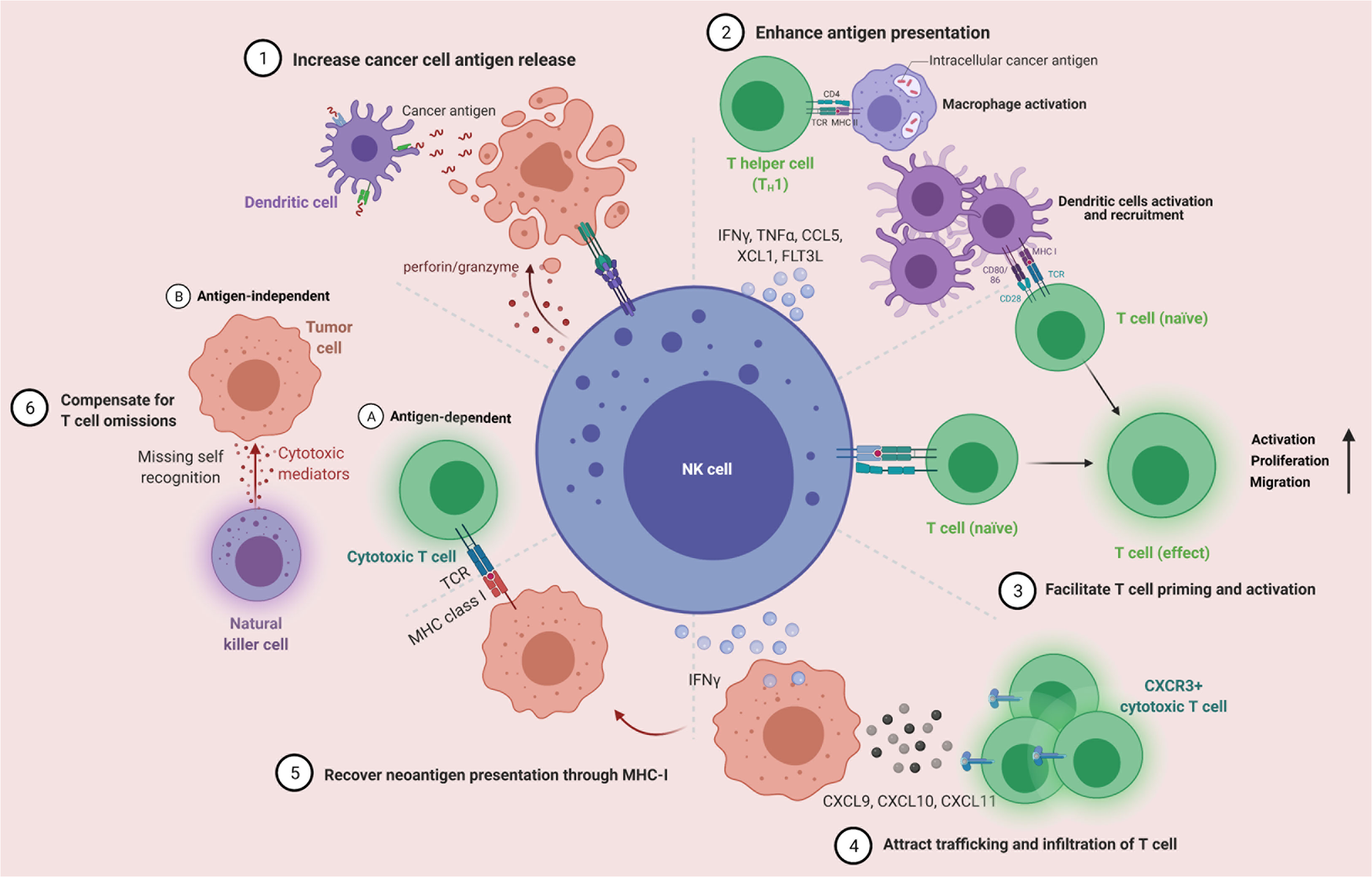The image is a detailed, scientific flowchart with a light pink background. At the center is a large, prominent blue circle labeled "NK cell." Surrounding this central circle are various smaller objects and illustrations that come in different colors such as blue, red, green, purple, and light auburn. Each of these objects is accompanied by descriptive text. The chart is organized into six steps: 1) Increase cancer cell antigen release, 2) Enhance antigen presentation, 3) Facilitate T cell priming and activation, 4) Attract trafficking and infiltration of T cells, 5) Recover neoantigen presentation through MHC class I, and 6) Compensate for T cell omissions. These steps and illustrations cover the entire flowchart from left to right, presenting a comprehensive visualization of some kind of immunological process, likely related to how NK cells and other immune cells interact with cancer cells. The chart is colorful, intricate, and aimed at summarizing complex biological mechanisms.